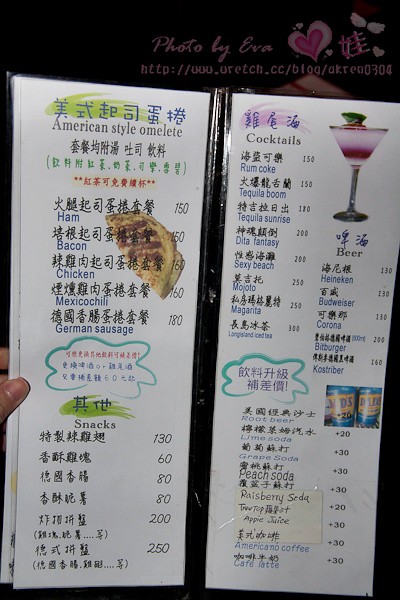The image captures a vertically-opened, black-bound menu with white pages, displaying offerings with a blend of Asian and English text. The left page prominently features the "American Style Omelet," listing additional ingredients that can be added. A hand, with the thumb and two fingers visible, is seen holding the page open.

Beneath the omelet section, there's a header titled "Snacks," featuring various items written in Asian script without English translations. Pricing is visible on the right-hand side; however, the currency is not explicitly identified.

The right page is divided into sections for "Cocktails," "Beer," and non-alcoholic beverages such as root beer and grape soda. Each cocktail listing includes English translations beneath the Asian characters.

Above these sections, the credit "Photo by Eva" is displayed in pink, accompanied by a heart and other small pink icons, and includes a link to the photographer's website.